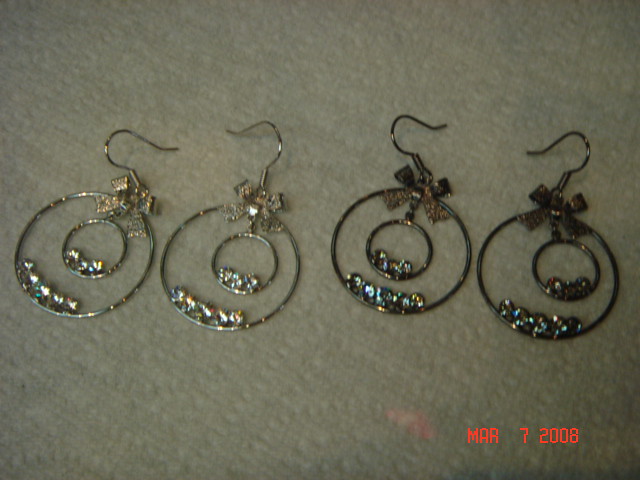The image showcases two sets of earrings arranged on a subtly textured green carpet, which has small holes indented into its surface. The date "Mar 7, 2008" is displayed in orange font in the bottom right corner. The earrings on the left are metallic silver with two concentric circles. The outer circle features five small, shining silver jewels resembling diamonds, while the inner circle contains three similar jewels. Each silver earring is adorned with a delicate metal bow just above the circles, leading to the hook. The earrings on the right mirror this design but are a black metallic color. They also have an outer circle with five black beads and an inner circle with three smaller black beads, complemented by a black bow at the base of the hook.